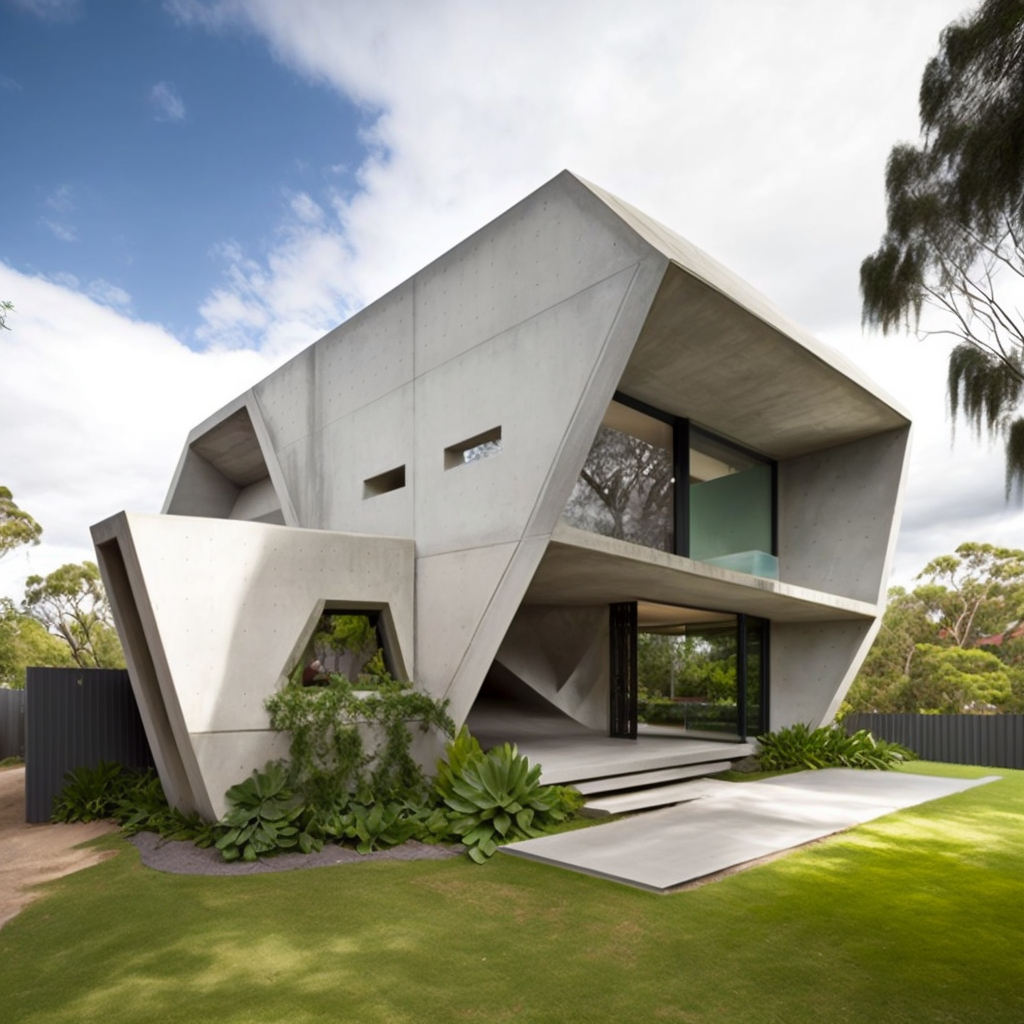This image showcases a highly modernistic, futuristic-looking house, constructed from concrete and characterized by its geometric design with predominantly 60-degree and 135-degree angles, reminiscent of structures in movies like "Logan's Run" and "Sleeper." The two-story house features an upper floor that is wider than the bottom story, with expansive windows. The top story showcases large sections of glass supported by black beams, creating a striking contrast against the white exterior. The front side of the house is divided by prominent seams, evidencing its panel-based construction. There is a balcony area jutting out from the upper story, also made of concrete.

The bottom floor of the house appears more open, with an archway providing access and two slits serving as windows. The entire structure is enveloped by a well-maintained, green lawn and minimal yet deliberate landscaping, including large succulents near the steps. There are two concrete steps leading to a small pad in front of the house. The property is enclosed by a gray fence, with additional trees and shrubbery providing privacy toward the rear. Overhead, the sky is mostly cloud-filled with patches of blue visible. Additionally, a tree is noticeable at the top right corner of the image, further enhancing the natural surroundings reflected in the house's large glass windows.